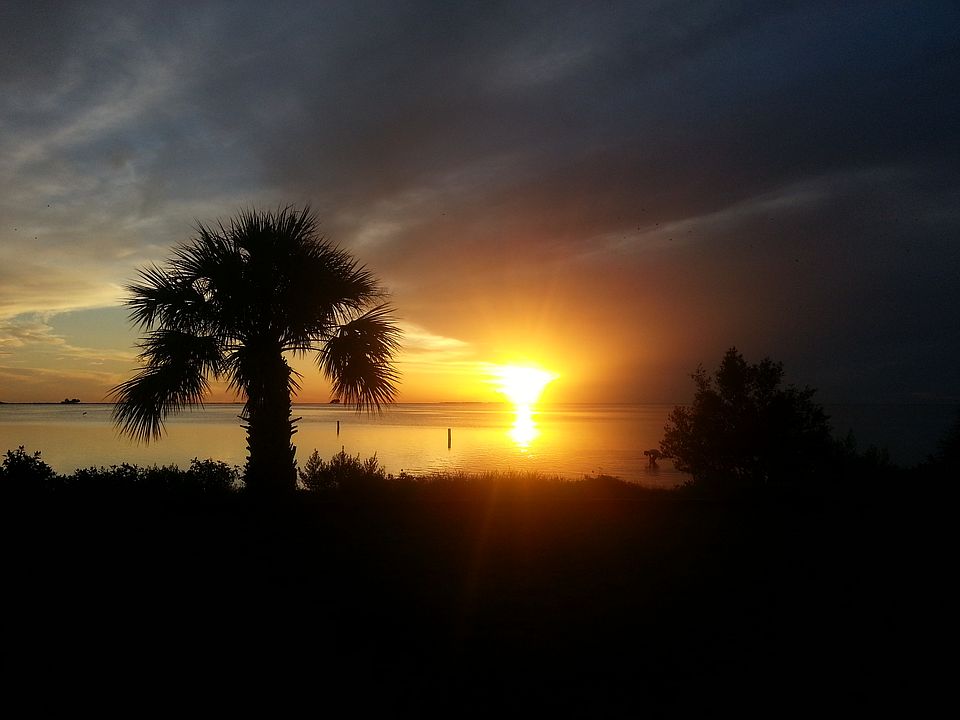The photograph captures the serene beauty of a tropical sunset over calm water. In the landscape-oriented image, the darkened foreground features the silhouetted outlines of a spiny palm tree on the left, low grass, and a bush on the right. Peeking between these natural elements are two posts protruding from the water and the faint silhouette of a person bending down near the shore, adding a touch of life to the tranquil scene.

The sky transitions from darkness in the upper-right corner to a lighter blue and gray towards the left. Wispy clouds float in the twilight sky, which is dramatically illuminated by a bright, almost-setting sun. The sun's brilliant yellow and orange hues reflect stunningly off the calm water, casting shimmering rays that stretch towards the viewer.

In the distance, small boats can be seen dotting the horizon, contributing to the photograph's peaceful ambiance. The overall impression is one of quiet, reflective beauty as day turns to night in a picturesque tropical paradise.